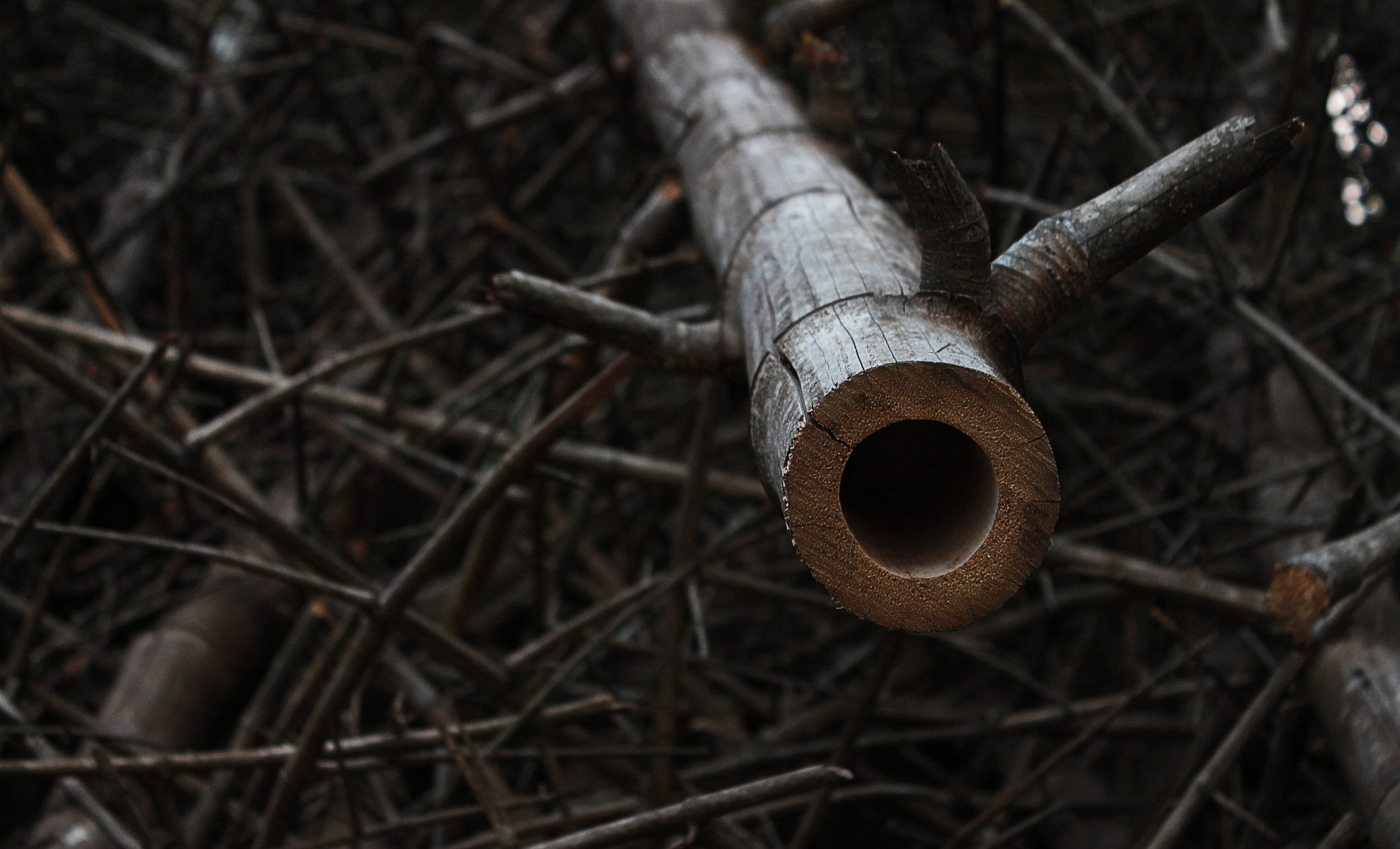This close-up image captures the hollow, cylindrical interior of what appears to be a tree branch or wooden log, likely cut cleanly with an electric saw. The log is dark brown with signs of cracks and broken branches along its sides. The view offers a side perspective, revealing the circular, hollow center that recedes into darkness. Surrounding the main log, the background is a busy, intricate pattern of numerous thin branches and logs in various shades of brown and gray. These branches extend in multiple directions, creating a complex and textured scene that suggests a natural environment cluttered with similar debris. The overall color palette is dominated by dark browns and grays, with patches of weathered, lighter brown bark suggesting slight decay or weathering.